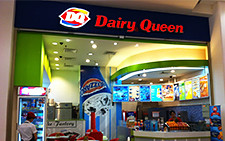The image depicts a small, blurry photograph of a Dairy Queen store, likely situated inside a mall due to its design and layout. At the top of the store, there's a dark blue or black background featuring the Dairy Queen (DQ) logo, which includes the white letters "DQ" against a red backdrop, accompanied by the distinctive blue and yellow swirl. To the right of the logo, the words "Dairy Queen" are illuminated in red neon lights. The store appears to be open, as seen through the lit interior. The menu is visible but indecipherable due to the blurred quality of the image, though its bright colors stand out. Inside, a person can be faintly seen standing at the counter in front of a register, and another individual, possibly an employee, is visible near a refrigerator wearing a hat and white shirt with their back turned. Additionally, a sign promoting Blizzards or another ice cream treat is noticeable within the store. The overall setting of the image is brightly lit and colorful despite the low resolution and tiny size of the picture.